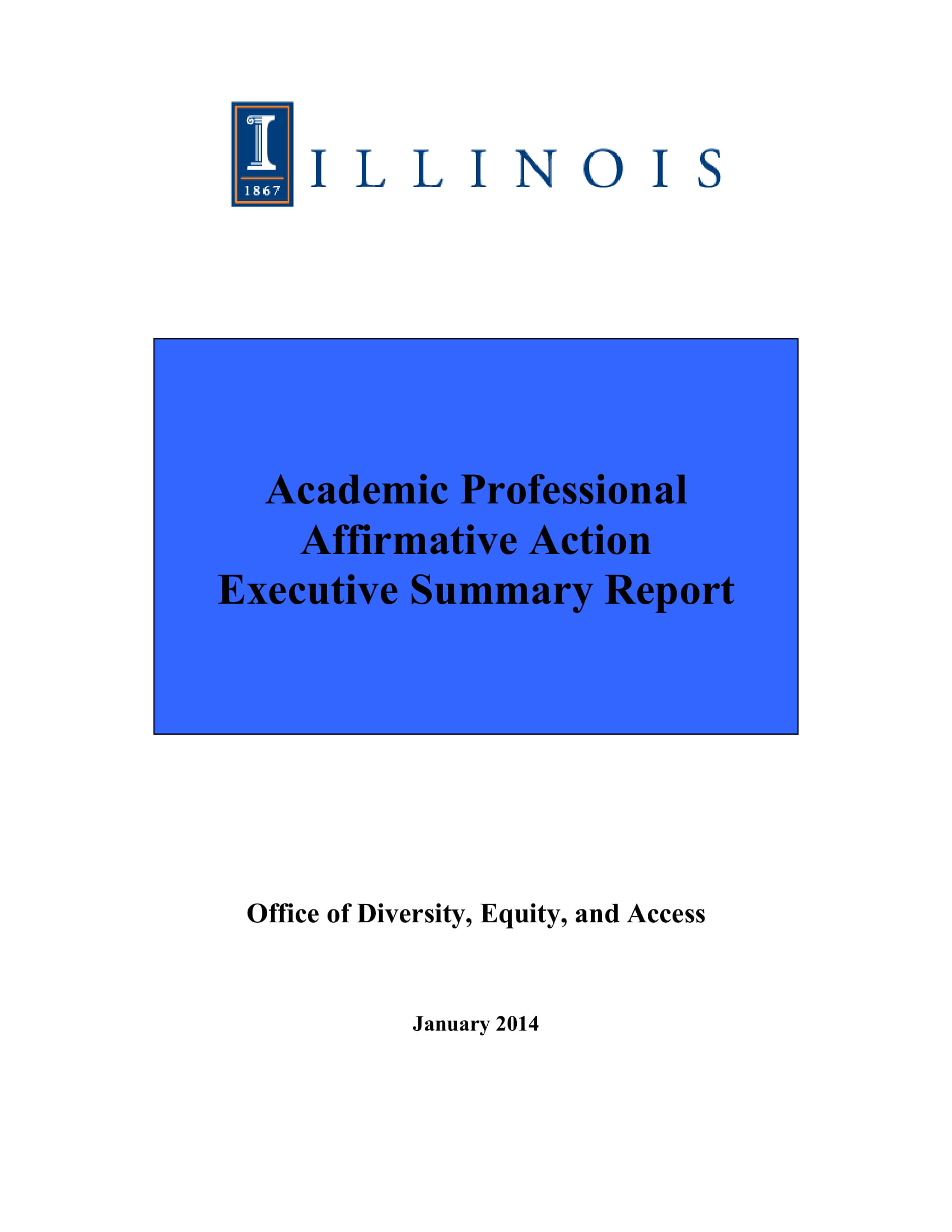The screenshot from the website displays the branding and key details of a document. At the top of the image, there's a dark blue rectangle prominently featuring the business logo. This logo comprises a smaller golden rectangle band inset within the dark blue background, accompanied by a stylized white eye resembling a Greek pillar. Below this logo, a gold line runs horizontally, creating a frame around the golden rectangle. Enclosed within this frame, the numbers "1867" are displayed, suggesting the founding year of the entity. The word "ILLINOIS" follows below, spelled out in bold, capital blue letters.

Continuing the composition, another dark blue rectangle appears with bold black text that reads: "ACADEMIC PROFESSIONAL," followed by "AFFIRMATIVE ACTION," and finally "EXECUTIVE SUMMARY REPORT," each on a separate line.

In the main section of the background, which is predominantly white, there is more pertinent information. Bold black text identifies a sub-header: "OFFICE OF DIVERSITY, EQUALITY, AND ACCESS." Further down in this white area, centered black bold text indicates "JANUARY 2014," denoting the document's publication date.

This detailed layout suggests that the screenshot captures the cover page of a report published in January 2014 by an Illinois-based institution, specifically focusing on the topics of academic professionalism, affirmative action, and executive summary insights provided by the Office of Diversity, Equality, and Access.